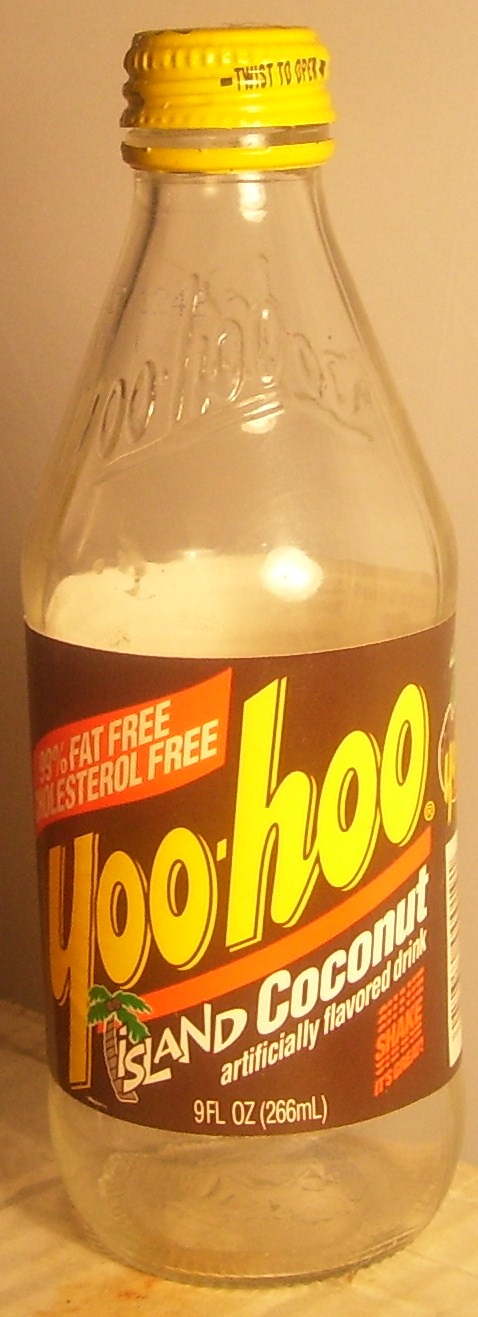This detailed, close-up color photograph depicts a drink bottle against a background featuring a light brownish wall and a yellowish, wooden-looking surface beneath. The entire image appears to have a yellow tint, possibly from a filter, giving it hues of yellow, brown, and orange. The bottle itself could be made of either glass or plastic and is topped with either a black or yellow cap, which bears an unreadable "Best Before" date in black text.

An embossed design decorates the upper part of the bottle, though it is not legible. The label on the bottle has a brown background with orange accents. At the center of the label is a yellow logo with the word "Yahoo" and an illustration of a palm tree. Next to this, in white text, the label reads "Island Coconut Artificially Flavoured Drink." Below that are the measurements "9 Fluid Ounces 266ml." The upper left corner of the label highlights the drink's health benefits, stating "Fat Free, Cholesterol Free." To the far right of the label, a small portion of either a barcode or a nutritional label is visible. Notably, the bottle appears almost empty, with little to no liquid remaining inside.